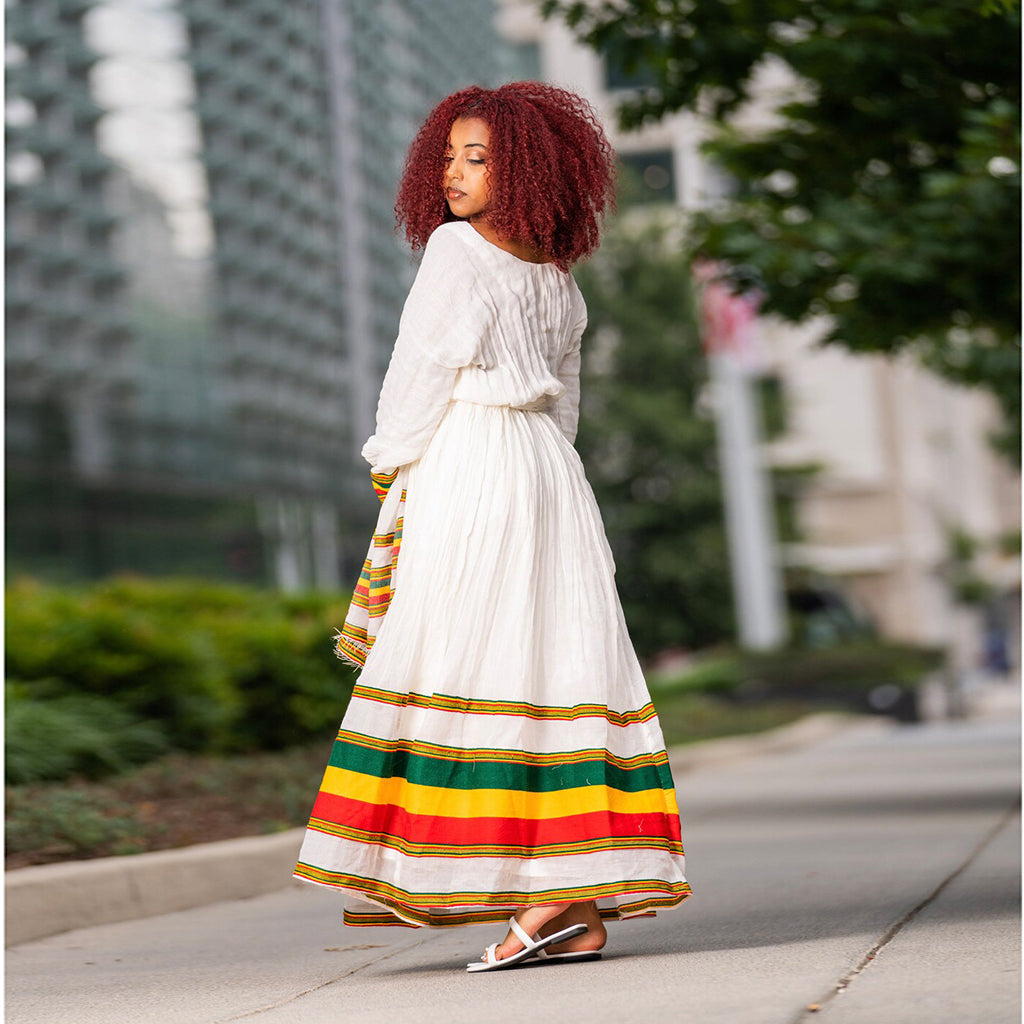A young African-American woman with medium-dark skin and striking red Afro hair is posing almost dreamily for a photo in the center of a bustling city scene. Her eyes are gently cast downward, nearly closed, as if lost in thought. She is dressed in a gracefully flaring white gown that transitions into a cascade of colorful stripes—gold, green, yellow, red, and more gold—starting from her knees down to the hem of the dress. She is wearing simple flat sandals and appears to be holding a shawl in her hands. The backdrop features a cityscape with tall, somewhat blue commercial buildings, flanked by lush greenery with bushes and trees. She stands on a gray sidewalk that borders a street, suggesting she's amidst the daily urban hustle and bustle, yet she exudes a calm, almost magical presence.